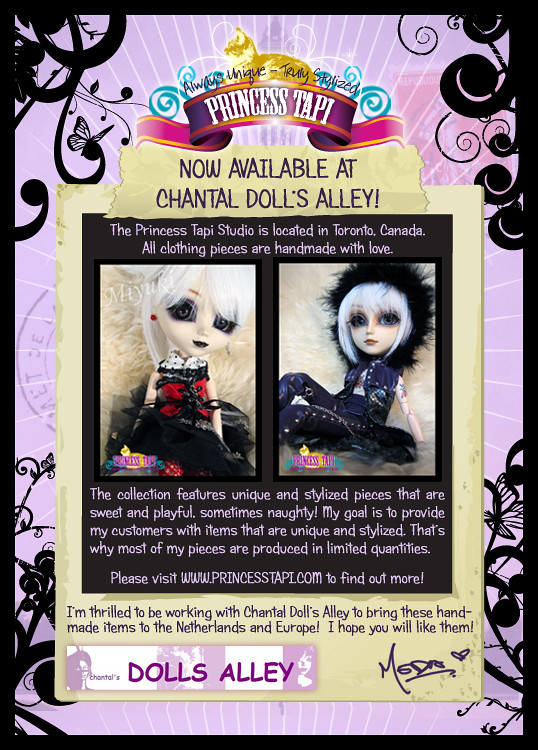This advertising poster captures the essence of the Princess Toppy brand with meticulous detail. Set against a pink and purple swirly background with elegant black, flowery curls and white lines at the borders, the centerpiece of the image prominently features "Princess Toppy" in bold white lettering over a luxurious purple ribbon. Below it, the text announces in capital letters, "Now Available at Chantal's Dolls Alley!" The poster provides a glimpse into the Princess Toppy studio, proudly located in Toronto, Canada, emphasizing that all clothing pieces are "handmade with love."

Central to the image are two striking dolls positioned horizontally side by side. Both dolls, with their unique, stylized appearances and white Hair, epitomize the brand's "sweet and playful, sometimes naughty" aesthetic. One doll is dressed in a red top and black skirt, while the other sports a cute jean outfit. The intricate designs of the dolls showcase the brand’s craftsmanship in creating limited quantities of unique and stylized pieces.

Accompanied by a heartfelt message from the creator, the poster expresses excitement about the collaboration with Chantal's Dolls Alley to bring these handmade items to the Netherlands and Europe. A call-to-action invites viewers to visit www.princesstoppy.com for more information, written in a charming pink or purple font. The poster concludes with "Dolls Alley" in all caps and a signature at the bottom right corner, merging both creative flair and a personal touch.